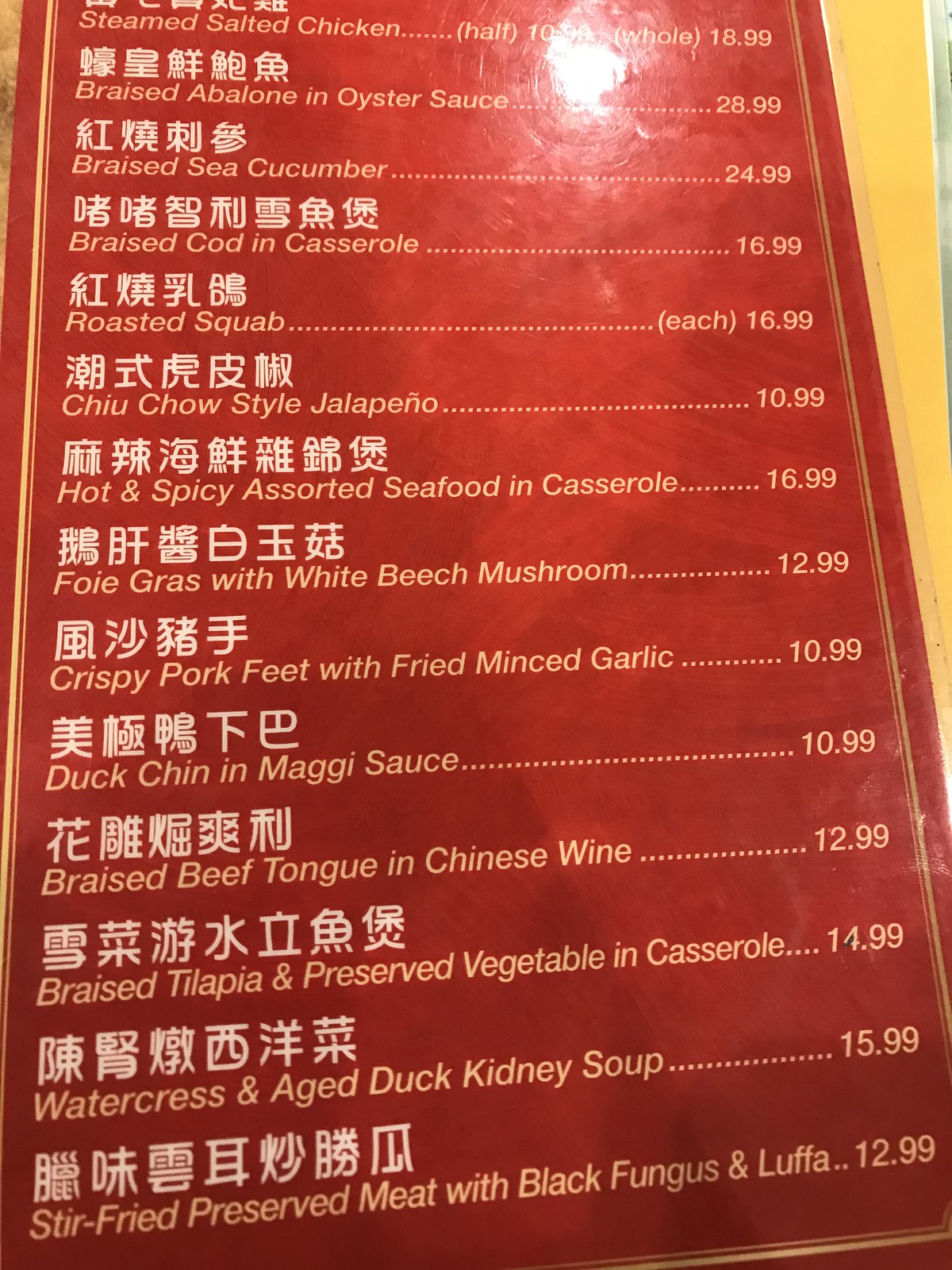This image features a detailed menu from a Chinese restaurant, elegantly designed with a red background and a gold border. The menu's text is written in a golden font against a yellow backdrop. A reflection of ceiling light is visible in the upper right-hand corner of the menu, adding a subtle highlight. The menu items are listed in both Chinese characters and English translations, offering an array of traditional and gourmet dishes, including:

- Steamed Salted Chicken
- Braised Abalone in Oyster Sauce
- Braised Sea Cucumber
- Braised Cod in Casserole
- Roasted Squab
- Chewy Chow Style Jalapeno
- Hot and Spicy Assorted Seafood in Casserole
- Foie Gras with White Beech Mushroom
- Crispy Pork Feet with Fried Minced Garlic
- Duck Chin in Maggi Sauce
- Braised Beef Tongue in Chinese Wine
- Braised Tilapia and Preserved Vegetable in Casserole
- Watercress and Aged Duck Kidney Soup
- Stir-Fried Preserved Meat with Black Fungus and Luffa

The design and presentation of this menu reflect the rich culinary heritage and attention to detail characteristic of authentic Chinese dining experiences.